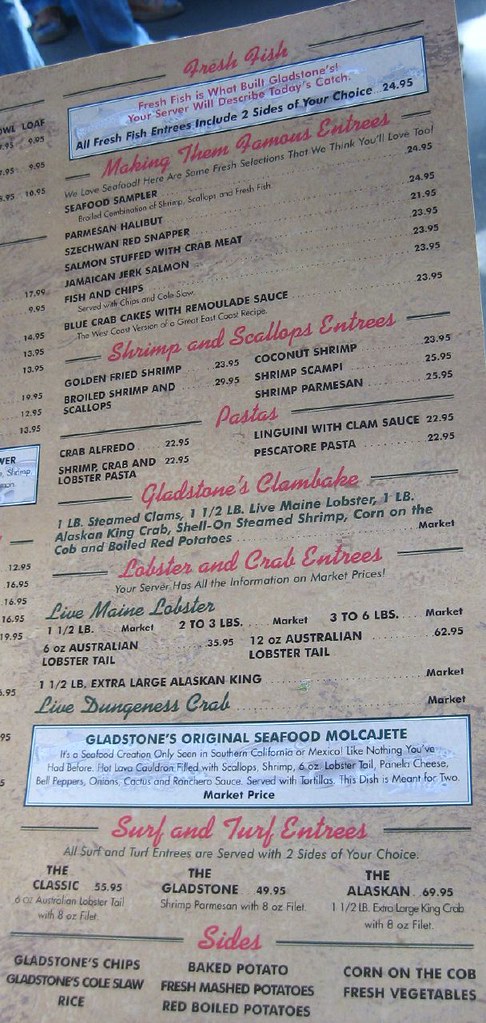This image depicts a segment of a restaurant menu, featuring a variety of fresh fish options. The headers, prominently displayed in red font, organize the menu's content. Below these headers, the specific items offered are listed in bold black font. Notably, special dishes are highlighted within a white box. The menu's background is a rich dark beige color, creating a warm and inviting appearance. The fresh fish offerings include a seafood sampler, Szechuan red snapper, and the classic fish and chips. Additionally, the menu includes seafood pastas, lobster, crab, and surf and turf entrees alongside a generous selection of sides such as chips, coleslaw, rice, baked potato, mashed potatoes, red boiled tomato, corn on the cob, and fresh vegetables. There are also tempting shrimp and scallop dishes. The restaurant may be called "Gladstones" as one of the headers reads "Gladstones Glam Bake." This partial view of the menu suggests that the restaurant boasts a wide array of culinary delights.